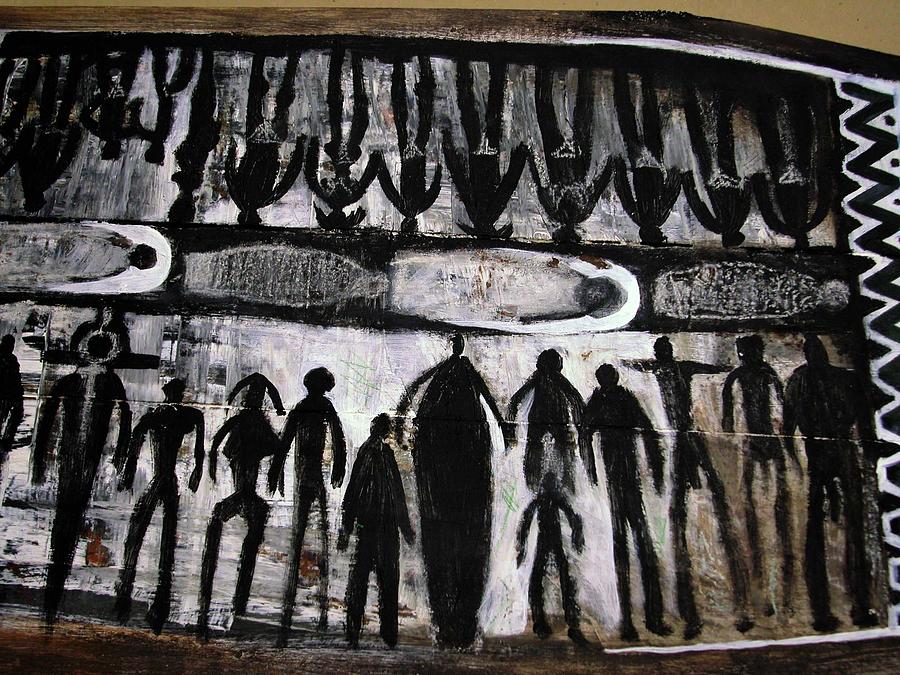This is a detailed color photograph of a black and white artwork painted on a piece of wood. The composition features a highly stylized and primitive depiction of numerous silhouetted figures. Along the bottom, a stripe of white provides the backdrop against which an array of people in various shapes, sizes, and arm lengths are silhouetted and filled in completely in black. The middle section showcases a horizontal row of what appears to be silhouettes of people lying down, potentially in coffins or beds, characterized by a black stripe with white smears across it. At the top of the painting, more silhouetted figures are rendered, except these are inverted, appearing upside down. To the far right of the image, a distinct black and white zigzag geometric pattern can be seen. The piece of wood on which this artwork is painted rests on a tan surface. The painting contains no distinguishable features, writing, animals, or man-made structures.